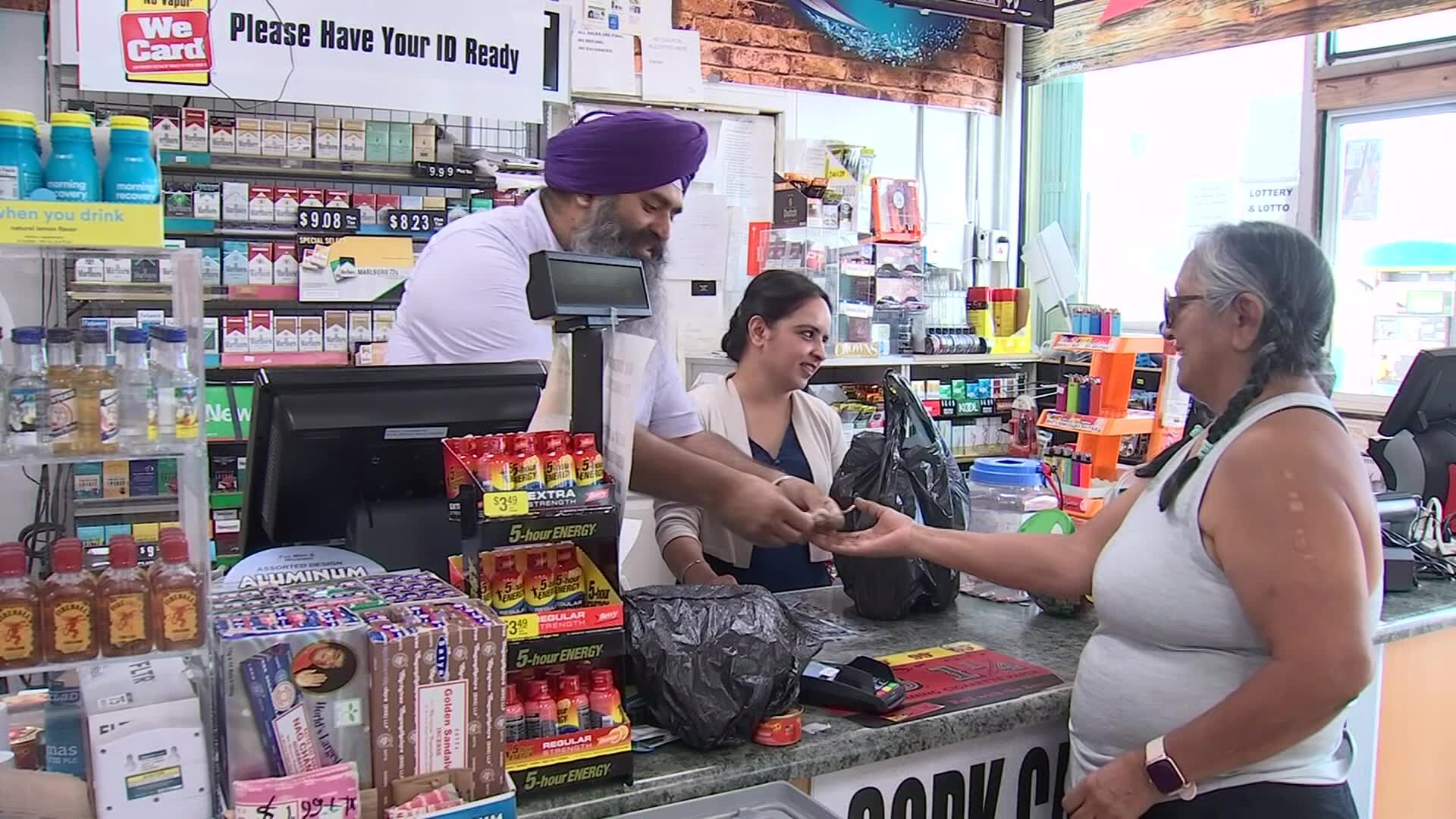In this detailed photograph taken inside a brightly lit convenience store during the daytime, we see a busy front counter scene. A young woman with short brown hair, wearing a blue sleeveless top over a white long-sleeve shirt, stands behind the counter, gazing towards the outside. Next to her, a man is assisting a customer; he is wearing a light purple shirt paired with a dark purple turban. This man is seen handing change to the customer, a woman with gray and black hair styled in pigtails, who is stretching out her hand to receive it. The customer is dressed in a gray tank top, black pants, and is notably sporting a pink Apple Watch.

The counter is cluttered with various items, including multiple rows of Five-Hour Energy bottles, along with a card machine and a small covered machine. Behind the counter, there are shelves displaying a multitude of cigarette cartons and boxes of incense. To the side, there is a clear glass display case containing small liquor bottles, against a backdrop of brick wall inside the store.